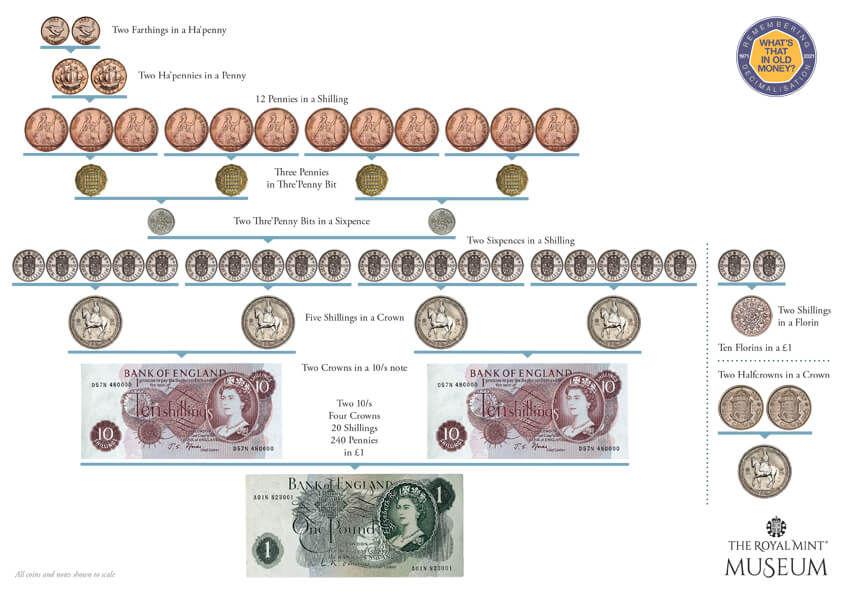This detailed infograph from the Royal Mint Museum, set on a white background, meticulously charts the various denominations of pre-decimal UK currency. At the upper right corner, a circular logo with blue text on a yellow background poses the question, "What's that in old money?" surrounded by white text referencing decimalization. The lower right corner bears the Royal Mint Museum logo and text in black.

The chart is arranged with images of old coins and banknotes beginning from the smallest denomination in the upper left corner. It starts with two farthings making a half-penny, two half-pennies making a penny, then progresses upward, showing how twelve pennies equate to a shilling, and three pennies to a threepence bit. It continues with conversions like two threepence bits making a sixpence, two sixpences forming a shilling, and five shillings equating to a crown. Further up the scale, four crowns make a ten shilling note, two ten-shilling notes make a pound, composed of 240 pennies.

The chart's illustrations include copper, silverish, and brownish coins, highlighting the varied materials used. The lower sections feature Bank of England banknotes adorned with the image of Queen Elizabeth II, available in different colors such as reddish-white and green, each with varying denominations including 10 S and 1 pound. The detailed visual aids on the chart delineate the transition from pennies and shillings up to crowns and pound notes, effectively capturing a historical snapshot of pre-decimal British currency.